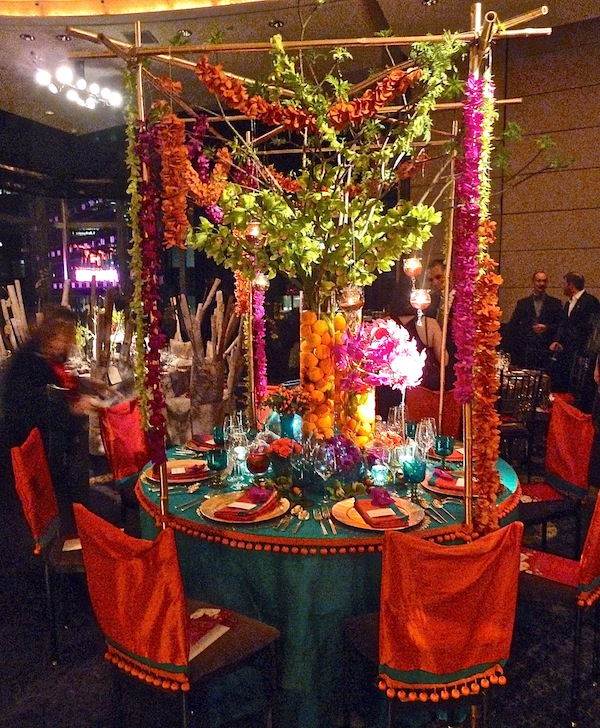In this vibrant and elaborate restaurant scene, a meticulously decorated table sits ready for a special occasion. The table, covered with a green cloth draped over its sides, is adorned with a mix of colorful elements. Red spheres and orange citrus fruits are arranged alongside green leaves, while purple petals flutter over the display. The chairs, wrapped in red fabric with tassels, line up symmetrically, and each setting includes red napkins, neatly arranged forks on the left, spoons on the right, and an assortment of glasses. Above, a canopy formed by pipes supports hanging floral garlands reminiscent of Hawaiian leis, accentuating the festive ambiance. In the background, men in black suits stand, some sharply visible, others blurred, adding to the formal atmosphere. The overall scene is bathed in vibrant colors including hints of pink, green, and light blue, with a spot of purple neon light casting a soft glow in the distance.